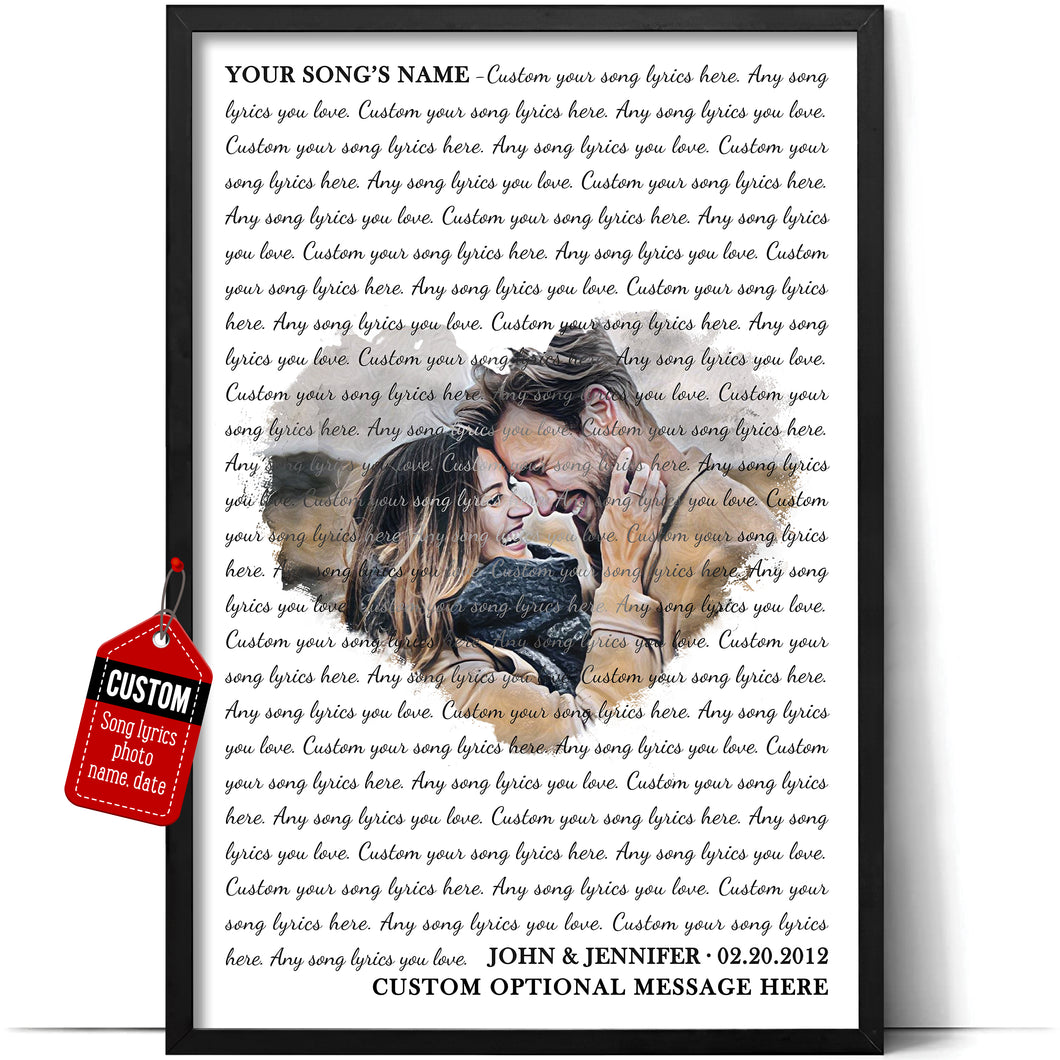The image features a vertically-oriented, rectangular framed poster with a sleek black border. At the center of the poster is a heart-shaped drawing of a man and a woman, in love, standing with their foreheads pressed together. The woman, positioned on the right, has long, dirty brown hair, and is wearing a light brown jacket and a blue scarf, her hands gently cupping the man's face. The man has shaggy brown hair, a thin beard, and a mustache, and is also dressed in a light brown jacket. Surrounding this affectionate scene is a series of cursive text scrolling vertically across a white background. The text provides a customizable template for personal lyrics, beginning with "Your Song's Name" at the top, followed by spaces to insert "custom your song lyrics here" for any special song lyrics. Further down, it displays names and dates, illustrated by the example "John and Jennifer, 02-20-2012," with an additional space for a custom message. A small red tag on the side highlights options for customizing the song lyrics, photo, names, and date, suggesting a thoughtful, personalized gift idea.